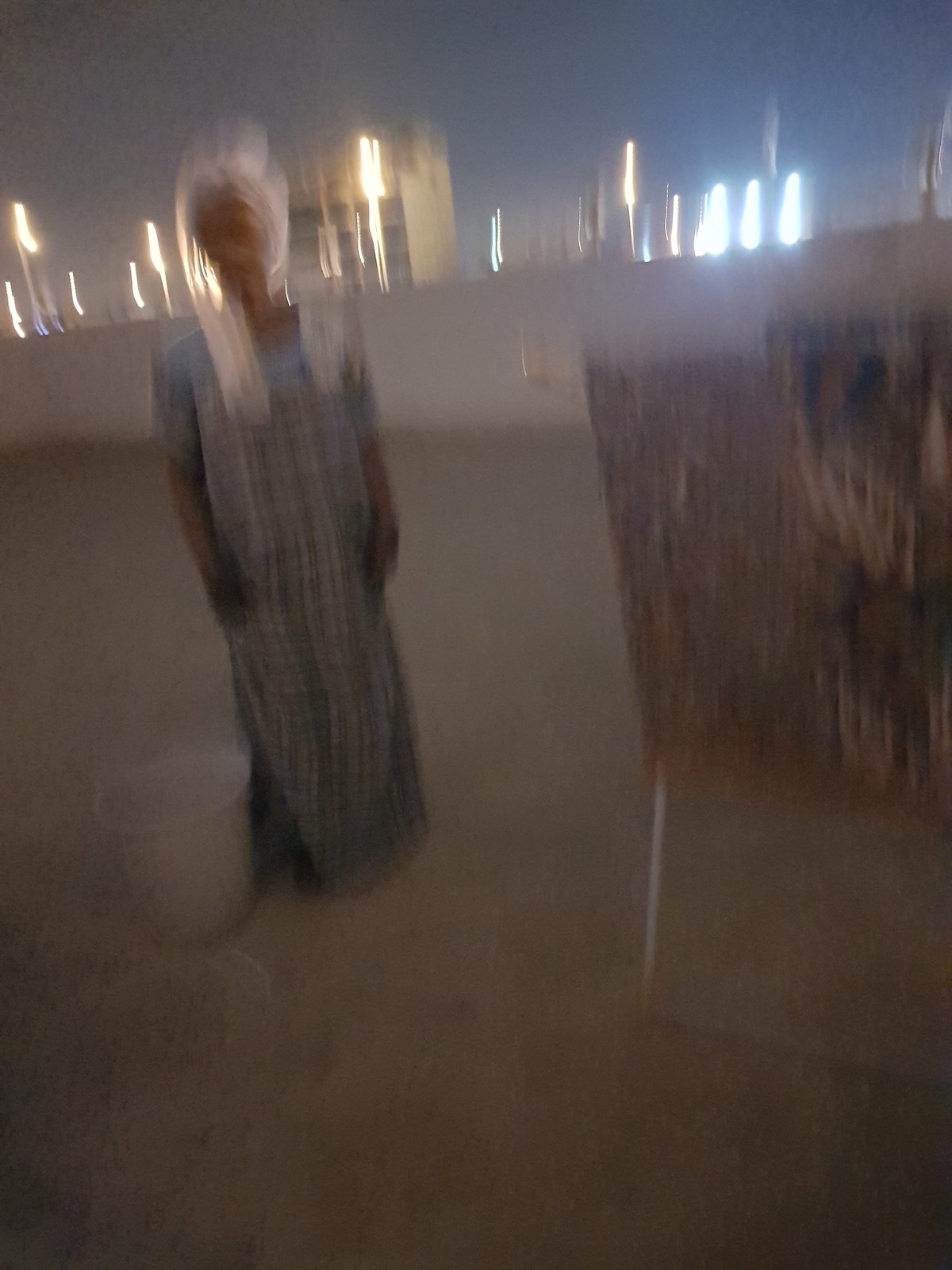In the image, a dynamic motion blur captures a person kneeling on a grey ground on the left side. The individual faces towards the camera and wears a white cloth covering their head and draping slightly down to the chest. Their attire consists of a grey dress adorned with vertical black stripes. To the left of the person, a white bucket is visible. The background features houses illuminated with lights, including yellow and blue hues. On the far left, there's a rectangular stand with white legs, displaying a mix of brown and white coloration. The combination of elements and the motion blur give the scene a sense of movement and vivid detail.